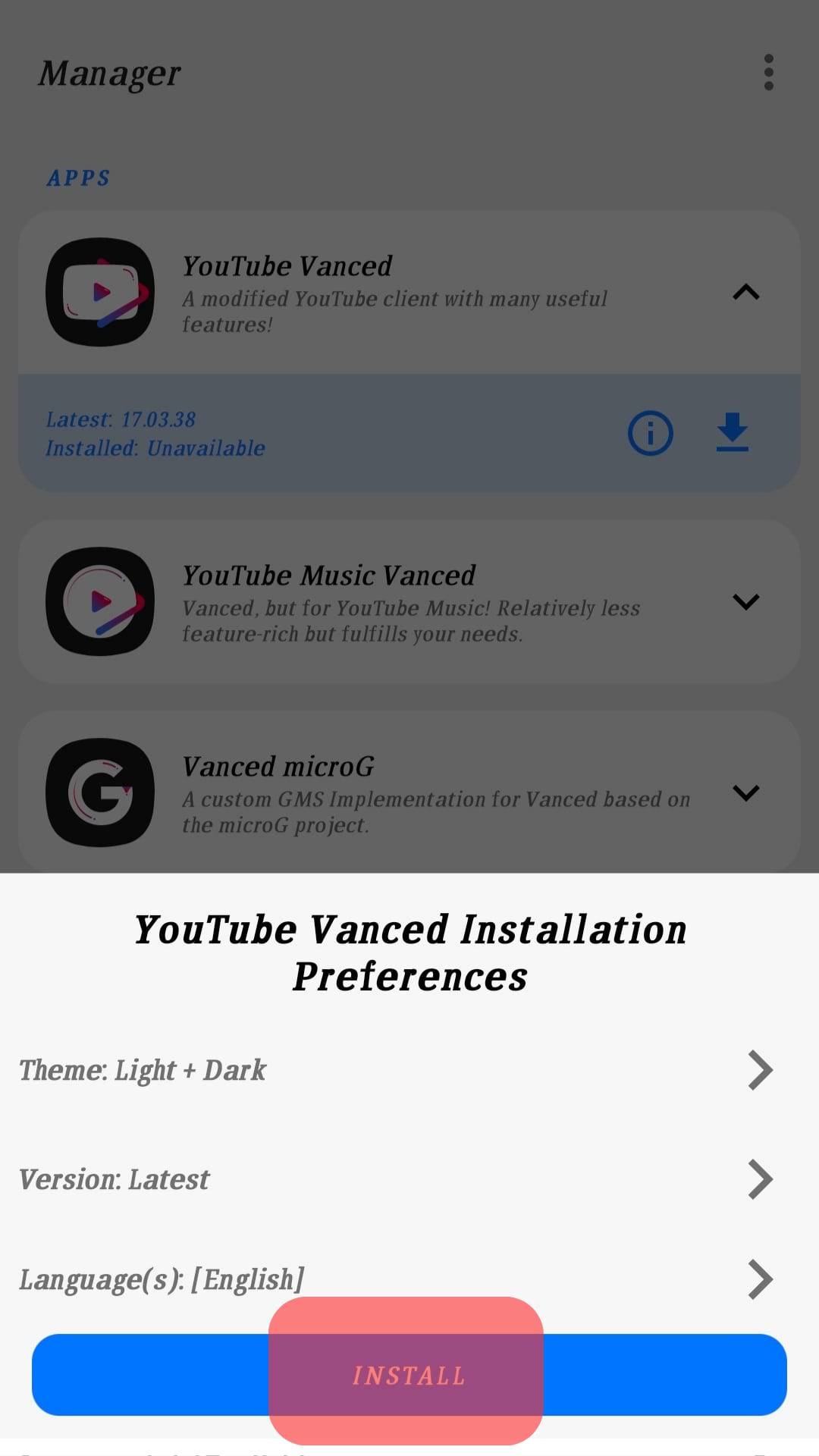The image displays a screenshot from what appears to be a mobile device, likely a smartphone, showcasing an app manager interface for a modified YouTube client. The screen is long and rectangular, resembling a typical smartphone display. 

At the top, the interface is muted and darkened, indicating that the options in this section are inactive and unclickable. The top section includes:
- The word "Manager."
- A category titled "Apps."
- A clickable area labeled "YouTube Vanced," described as a modified YouTube client with numerous useful features.

Below this, there are several inactive options:
- "Latest" followed by numerical values.
- "Installed" marked as unavailable.
- An "Information" button.
- A "Download" button.

Following this, there is another category for "YouTube Music Vanced" and one for "Vanced MicroG," which is described as a custom GMS implementation for Vanced based on the MicroG project.

The active portion of the screen is highlighted and slightly lower. It is a white box labeled "YouTube Vanced Installation Preferences." This section allows for interaction and contains several configuration options with directional arrows for more information:
- "Theme" with options like light and dark.
- "Version," showing the latest version.
- "Languages," currently set to English.

At the bottom of this section, there is an "Install" button prominently highlighted in red on a blue banner bar, indicating that it is clickable and ready for user interaction.